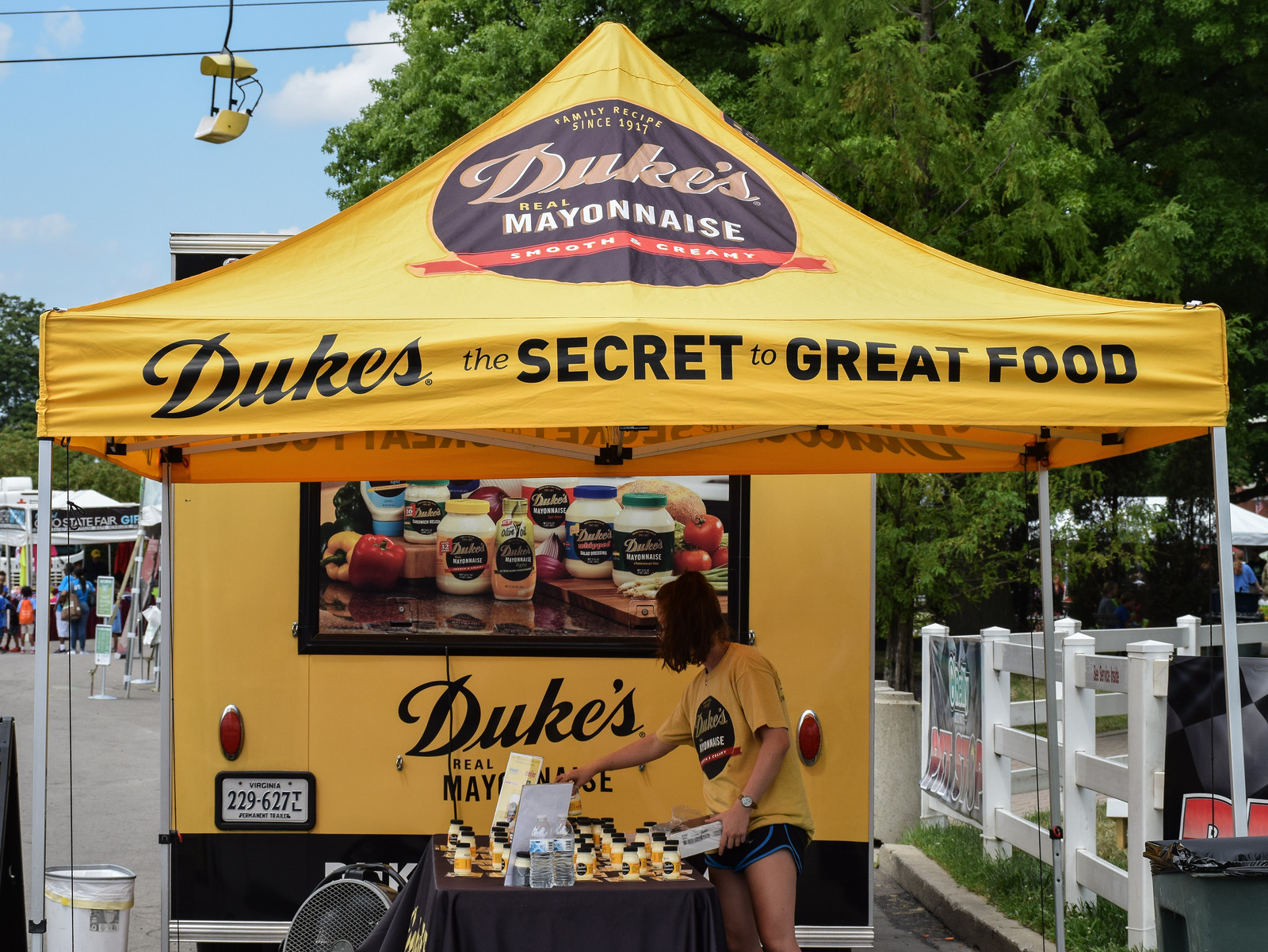This color photograph, in landscape orientation, captures a lively outdoor event, featuring a prominent yellow Duke's Mayonnaise pop-up canopy tent. The canopy is adorned with a round logo at the top, stating "Duke's Real Mayonnaise, smooth and creamy" against a black circular background, and the words "Duke's, the secret to great food" emblazoned along the top edge. 

Located under the tent is a young woman with short brown hair or in a ponytail, wearing a yellow Duke's Mayonnaise t-shirt and black and blue shorts. She stands near a black tablecloth-draped table scattered with jars of Duke's Mayonnaise, busy arranging items. 

Directly behind the tent is a Duke's Mayonnaise truck with a Virginia license plate (229-627-TL) featuring an advertisement with images of mayonnaise jars accompanied by tomatoes and peppers. A floor fan pointed upwards and a trash can are positioned near the legs of the tent. 

To the right, a white vinyl fence adorned with unreadable signs stretches out with a backdrop of trees and a clear sky. The event appears well-attended, with fair patrons seen near other tents in the distance. Above, there’s a glimpse of a lift system, perhaps a monorail, with no current passengers. The overall style of the photograph is representational realism, portraying a vivid, bustling scene at this fair or festival.